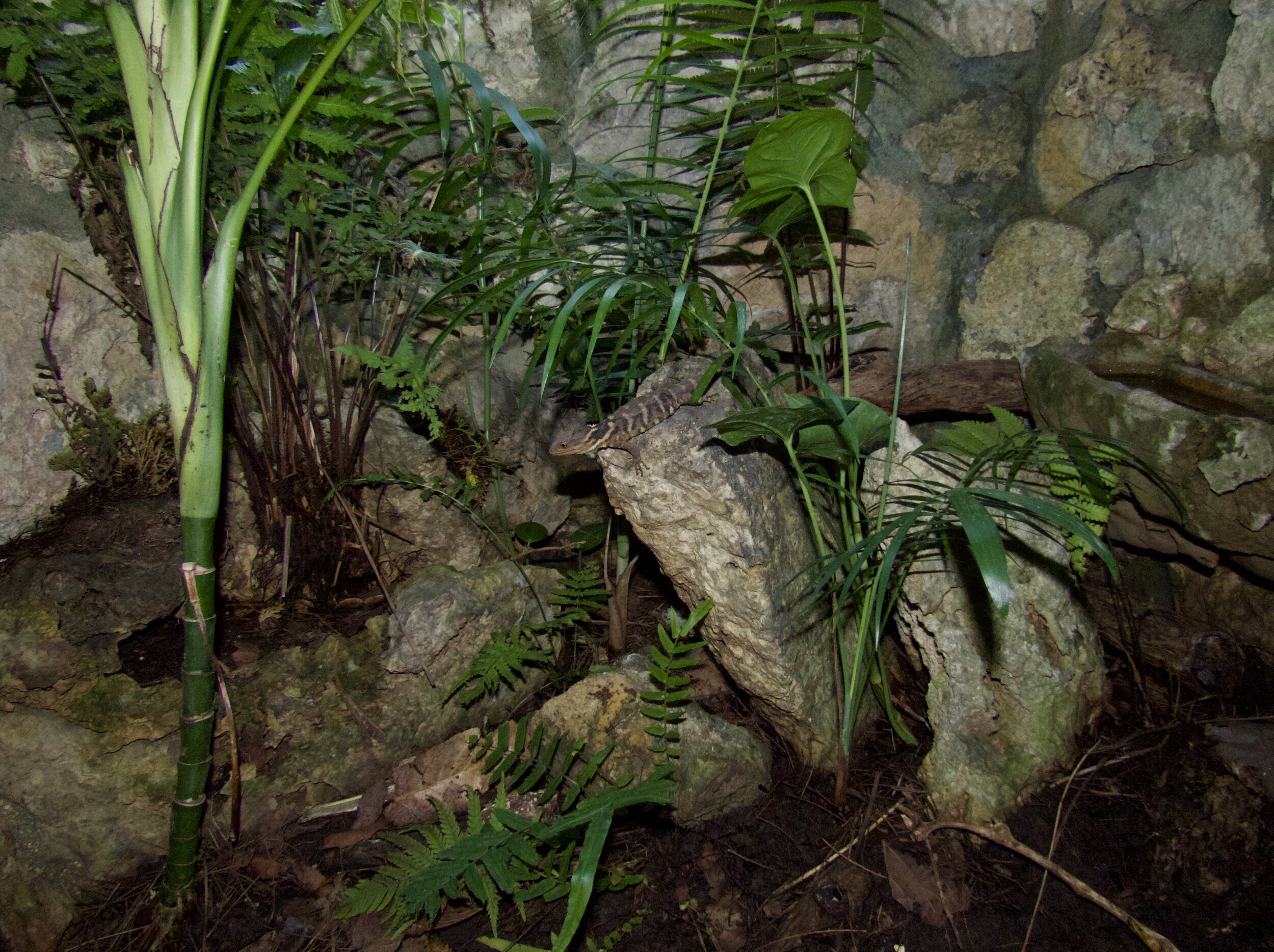The image captures a serene outdoor scene featuring a natural arrangement of elements. Dominating the foreground are four sizable, light gray rock formations surrounded by clusters of dark green leaves. These leaves are nestled among a few thin, tan branches. At the base of these rocks lies a layer of brown dirt or mulch, interspersed with several green leaves sprouting up from the ground.

To the left of the image, a vertically standing green stalk splits into multiple vines, contributing to the lush appearance of the scene. Additionally, a series of dark brown branches laden with dark green leaves can be seen in the background, blending with the overall verdant theme.

Completing the scenery is a backdrop of rocky terrain, predominantly colored in various shades of light and dark gray, adding texture and depth to this tranquil outdoor setting.